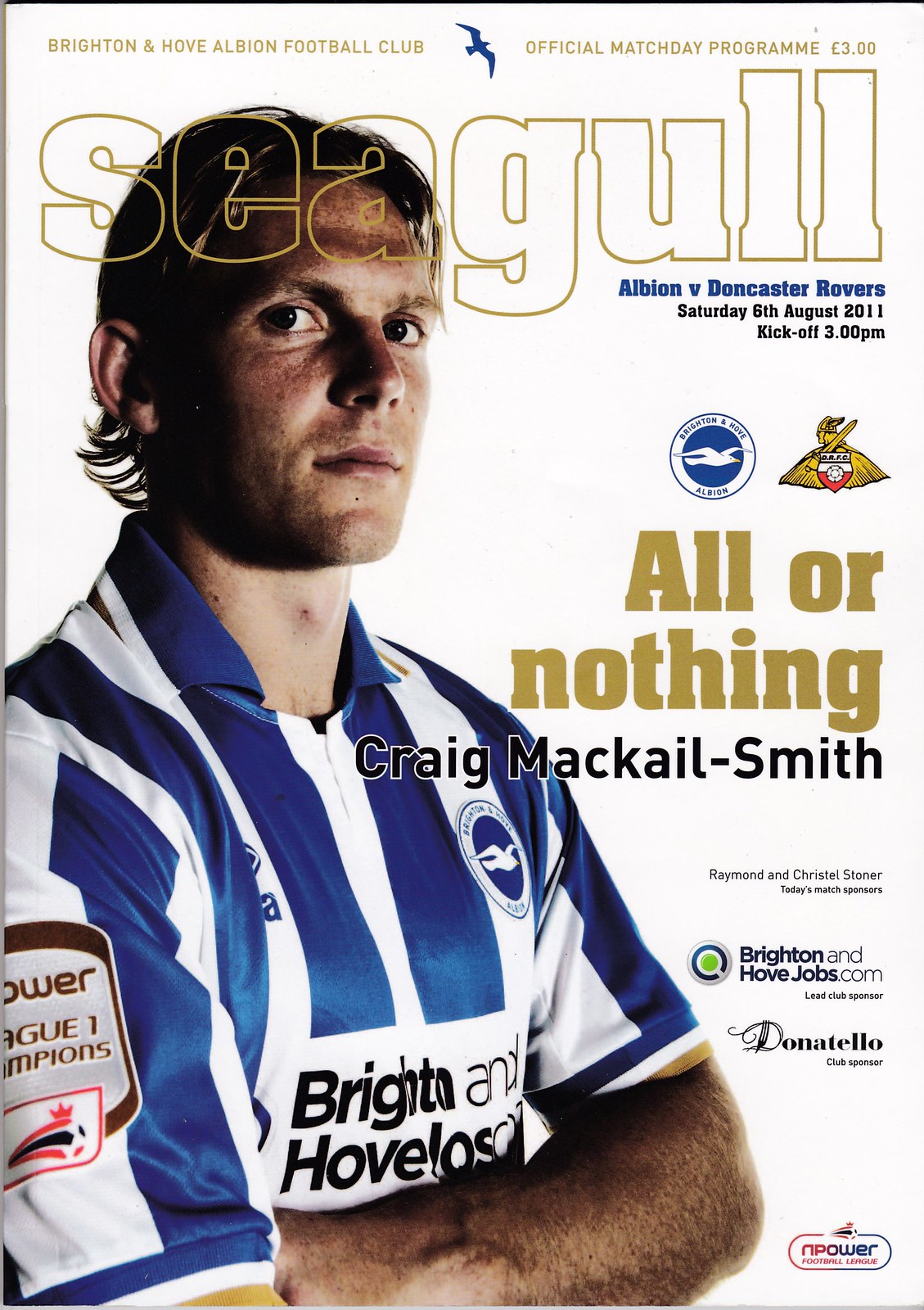This is a vertically aligned magazine cover for "Seagull," featuring a white background with the title "Seagull" in large, outlined white letters with a gold border. At the top in small print, it reads "Brighton & Hove Albion Football Club, official match day program, three pounds," accompanied by a blue seagull logo. 

Prominently positioned on the left side of the cover is an image of Craig Mackel-Smith, a soccer player from Brighton & Hove Albion Football Club. He is shown wearing a blue and white vertically striped jersey with a badge on his right arm and the club's name partially visible on his chest. With short blondish-brown hair and a serious expression, he looks slightly to the left, engaging the viewer.

Below the title, in blue print, it says "Albion versus Doncaster Rovers," followed by "Saturday, 6 August 2011, kickoff at 3 p.m." in black print. 

In the center of the cover, the phrase "All or Nothing" appears in bold gold letters, with "Craig Mackel-Smith" written in black underneath, partially overlaying his chest.

Down the right side of the cover are the logos of several sponsors including Raymond and Crystal Stoner, Brighton & Hove Jobs.com, Donatello, and Npower.